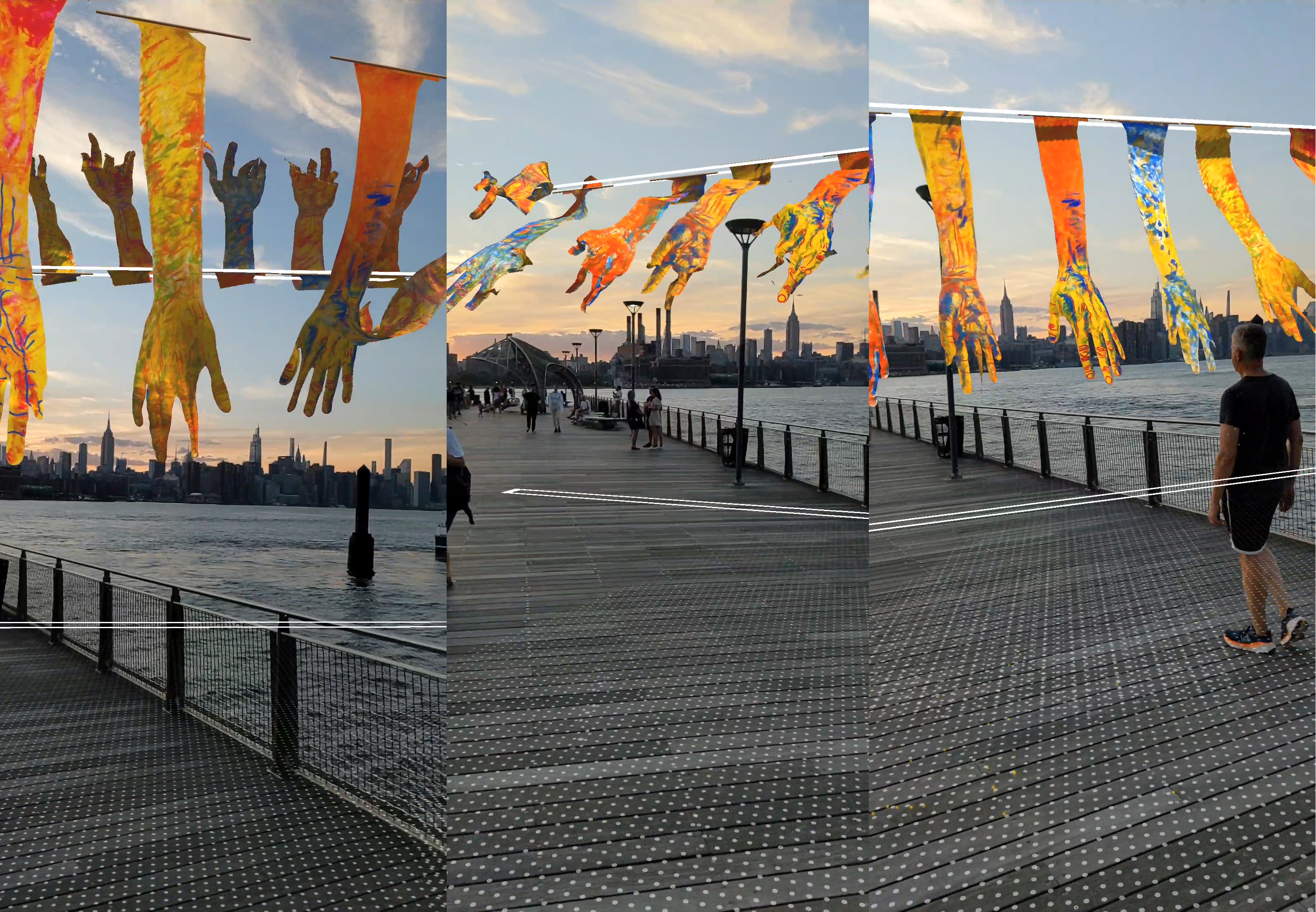The image is a composite of three vibrant photographs taken either just before sunrise or sunset, showcasing a unique art installation featuring long, ornamentally painted gloves hanging from clotheslines. Each photograph captures a different aspect of this scene:

1. The left photo prominently features a body of water, with the gloves gracefully suspended against a backdrop of a blue sky transitioning to twilight, dotted with some clouds.
2. The middle photo focuses on a gray metal dock bustling with people, and these beautifully colored gloves are seen hanging over the dock’s edge. The dock is lined with a rope fence, adding to its maritime feel. 
3. The right photo adds a touch of human presence with a middle-aged man in black shorts walking away from the display. The backdrop includes an urban skyline with tall buildings, hinting at a large city, potentially New York or Chicago.

The gloves themselves are striking, adorned with yellow, orange, and blue splotches, creating a vivid and whimsical pattern that stands out against the structural elements of the pier. In some images, the gloves appear to be animated by the wind, making them rise as if hands are holding them. Overall, this artistic display merges natural beauty with urban life in a captivating visual narrative.